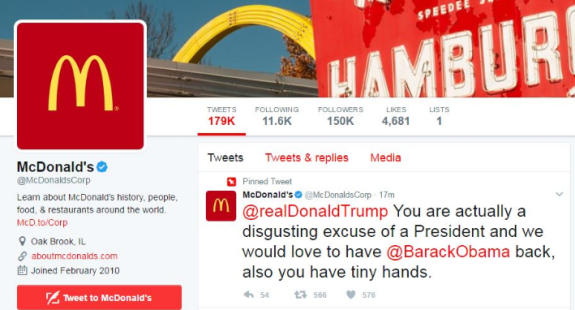This is the Twitter profile for McDonald's. The header image displays what appears to be the original McDonald's location, featuring the iconic golden arches and a prominent red sign that reads "Hamburger." The profile's avatar is red with the signature golden arch "M" logo.

The McDonald's Twitter account, under the handle @McDonaldsCorp, has tweeted 179,000 times. It boasts a follower count of 11.6 thousand and follows 150,000 accounts in return. The profile has received 4,681 likes and is listed once. The account is verified and lists its location as Oakbrook, Illinois. The bio includes a link to the official website, AboutMcDonalds.com, and notes that the account joined Twitter in February 2010. Below the bio, there is a red "Tweet to McDonald's" button.

On the right side of the profile, there is a pinned tweet from McDonald's posted 17 minutes ago. The tweet addresses former President Donald Trump, stating: "You are actually a disgusting excuse of a president and we would love to have @BarackObama back. Also, you have tiny hands." This tweet has garnered 566 retweets and 576 likes.